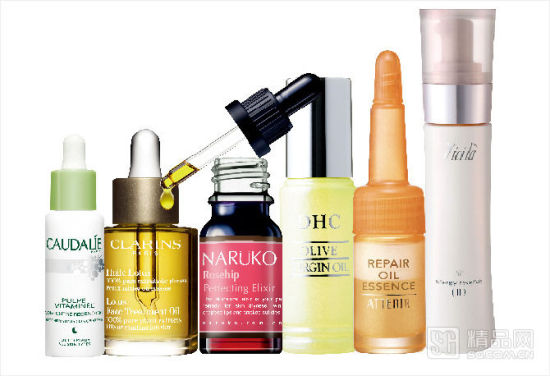This image showcases a variety of skincare products arranged on a white background, although the image quality is pixelated, making some text harder to discern. Starting from the left:

1. The first product is a slender white bottle with a vibrant green top. It is equipped with a dropper applicator. The bottle features green text that reads "Caudalie," though the smaller text beneath is unreadable due to pixelation.

2. Next, there is a wider clear bottle filled with a golden amber liquid. It has a bronze cap and a white dropper visible through the glass. The text on the bottle reads "Clarins."

3. The third item is a dark container with a red label that says "Naruko Rose Hip..." followed by additional text that is too pixelated to read clearly. The container’s cap has been removed, exposing the dropper which contains a similarly golden amber liquid with a droplet hanging off the tip. The top of the dropper is black.

4. To the right is a cylindrical container in a yellowy green hue. It has a silver, possibly squared, cap. The text on the bottle includes "HC Olive Virgin Oil," but the rest is indistinguishable.

5. The following product is an orange bottle with an orange cap that appears to feature some sort of dispensing tip. It is labeled "Repair Oil Essence."

6. Lastly, there is a large white bottle with a dual-colored cap. The top part of the cap is clear, revealing an interior that is pink, orange, or brown, and the base of the cap is silver. The text on this bottle is too pixelated to read clearly.

Despite the image’s pixelation, these details collectively portray a diverse assortment of skincare products, each with its unique packaging and design characteristics.